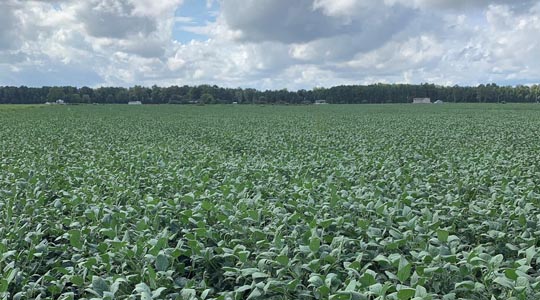This image captures an expansive, lush, green field that stretches across the entire foreground, densely covered with short, bushy plants whose exact type is not identifiable but may be soybeans or another type of vegetation. The foliage is thick and uniform, completely obscuring the ground beneath and extending uninterrupted for about two-thirds of the image. In the background, a number of scattered farmhouses and clusters of trees are visible, providing a picturesque rural setting. The sky overhead is a mix of stormy-looking clouds with patches of blue, suggesting a potentially variable but primarily cloudy day. The verdant scene is embraced by what seems to be a warm, outdoor atmosphere.